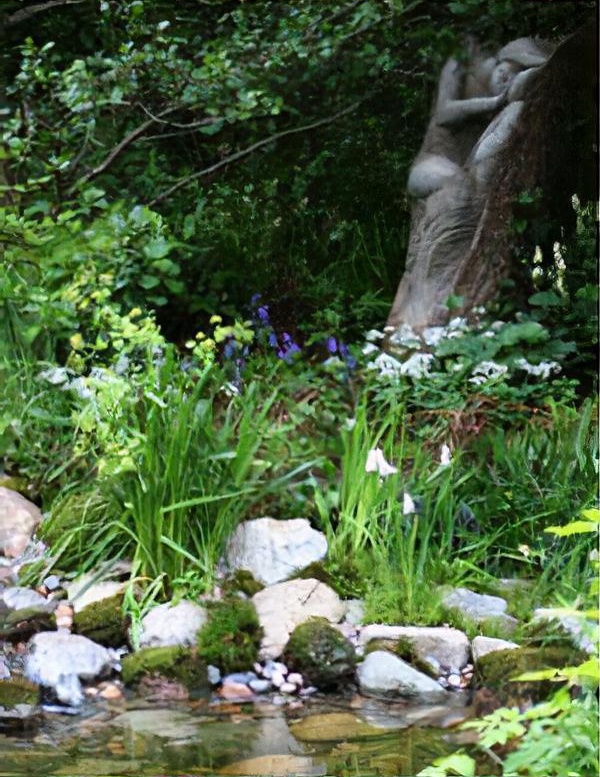The image captures a serene outdoor scene featuring a small creek meandering through an area dotted with various-sized rocks, including some covered in moss. Tall grasses and a variety of flowers, including purple, yellow, and white blooms, add vibrant splashes of color to the landscape. Clear water in the creek reflects the rocks beneath, enhancing the tranquil ambiance. Trees surround the area, with branches extending outwards, some of which intriguingly resemble a statue. Upon closer inspection, in the right-hand corner, there appears to be a form resembling the side and arm of a naked woman, possibly made of stone. This ambiguous shape could either be an artful statue or simply a uniquely contorted tree trunk.